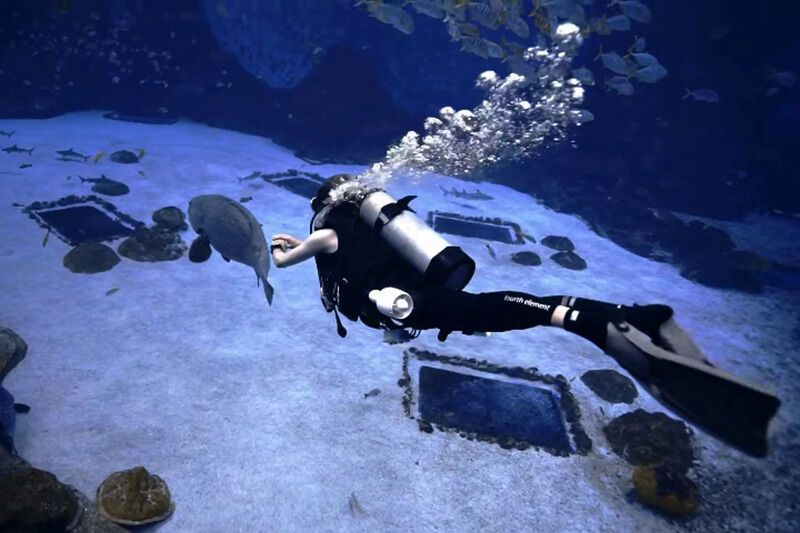This color photograph captures an underwater scene featuring a scuba diver, possibly a woman, discernible by the slenderness of their arms, fully equipped with a large oxygen tank and black sleeveless scuba suit. The diver, outfitted with flippers and possibly a wristwatch, is swimming through a vibrant marine environment thick with aquatic life. Bubbles trail from her oxygen tank, suggesting heavy breathing, as she maneuvers over a sunken ship blanketed in sediment and marine growth. The wreck, adorned with windows, is nestled near large coral formations, providing a home to diverse sea creatures, including turtles climbing over its surface. A prominent fish swims alongside the diver, while a school of approximately 30 fish drifts above. In a particularly striking detail, baby sharks are visible in the background, adding to the dynamic and bustling underwater tableau.